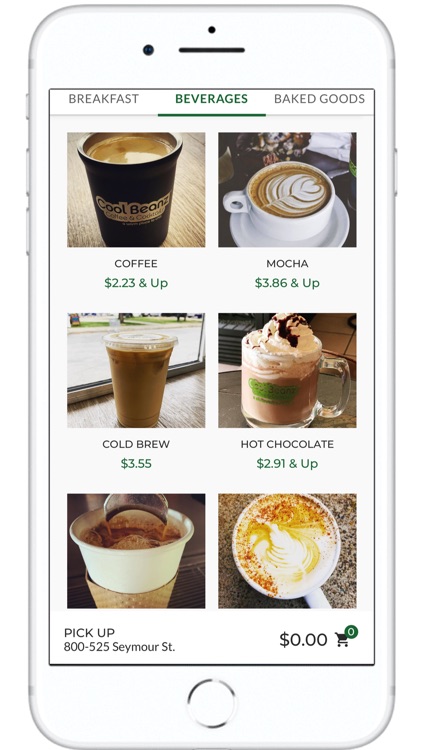A detailed image caption for the described scenario could be:

"This image captures a screenshot from a white cell phone, showcasing a menu for a coffee shop's offerings. The phone, identifiable by its left-side buttons for power/silencing and volume control, and a right-side button likely for power, displays a screen divided into categories: 'Breakfast', 'Beverages' (underlined in green), and 'Baked Goods'. Below these categories, six images arranged in a 2x3 grid present different items. The top-left item is labelled 'Coffee' priced at $2.23 and up, beside 'Mocha' priced at $3.86 and up. The middle row features 'Cold Brew' for $3.55 and 'Hot Chocolate' for $2.91 and up. The bottom row, partially cut off, includes options with a 'Pick-Up' notice for Seymour Street. The menu is vibrant and clearly structured, making it easy for users to navigate their beverage choices."